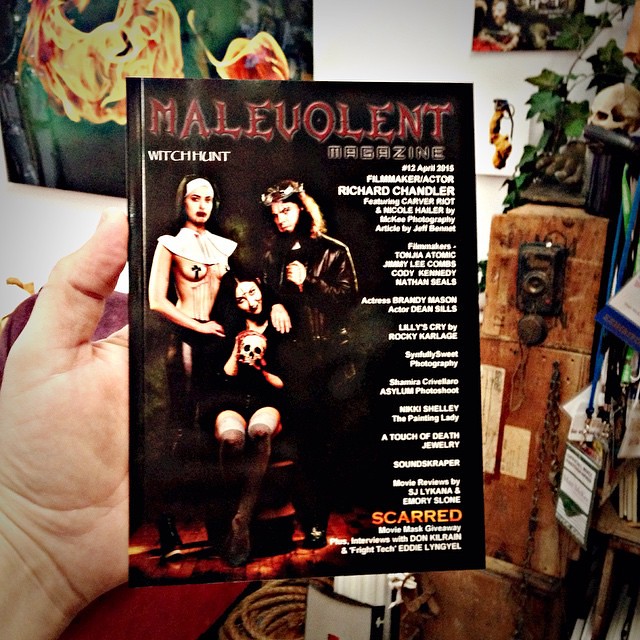This is a detailed color photograph depicting a square-format magazine cover being held by a person's left hand. The magazine, named "Malevolent," features its title boldly in red gothic letters atop a solid black background, with "Witch Hunt" written underneath in white. On the left side of the cover, three gothic figures are prominently displayed: a man with long brown hair and a beard wearing a black leather coat and some form of crown; a woman with long dark hair, red lipstick, a white collar, and white tape crossed over her breasts, with blood dripping down her chest; and another woman with short dark hair holding a skull, her hands smeared with blood. The right side of the cover is filled with white text detailing the magazine's contents: "Witch Hunt Magazine, Number 12, April 2015," featuring articles by McKee Photography and Jeff Bennett, and highlighting filmmakers Tanjia, Atomic, Jimmy Lee Combs, Cody Kennedy, Nathan Seals, actress Brandi Mason, actor Dean Sills, and "Lily's Cry" by Rocky Carlage. The background of the image displays various antiquities, books, and posters, contributing to a gothic and representational realism style.